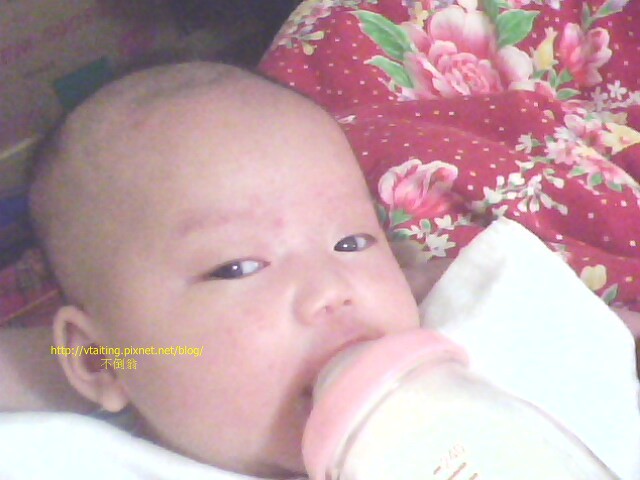The photograph depicts a very young newborn baby with striking brown eyes, looking directly up at the camera. The baby is lying on its back, comfortably positioned on a soft surface. A partially visible red floral design blanket is situated to the right of the baby's head. The baby is either wrapped in a white blanket or wearing a white garment that peeks above its shoulder. A clear, transparent baby bottle with a pink rim lid is in the baby's mouth, indicating that the baby is feeding on milk, as the bottle contains a white liquid. The setting appears to be indoors, given the controlled lighting and visible objects. In the bottom left corner of the image, there is a website link displayed in yellow text: "http://vtaiting.pixnet.net/blog/" followed by some Asian characters, suggesting the baby's possible Asian descent. The image is square, with the baby slightly positioned to the left, and the floral blanket prominently in the top right corner. The overall color palette includes hints of burgundy, pink, green, magenta, white, black, beige, and yellow.